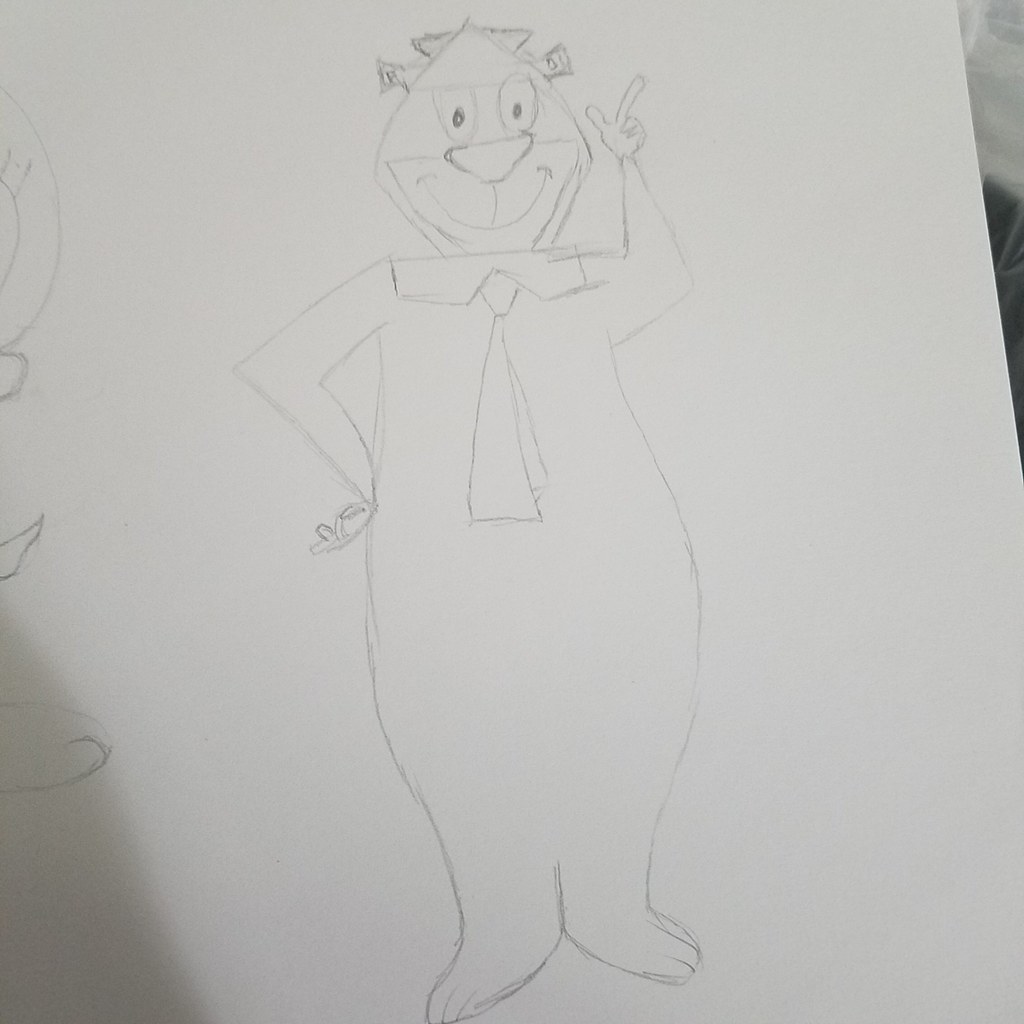This black and white photograph captures a child's line drawing rendered entirely in pencil. The drawing features a cartoon character resembling Fozzie Bear from the Muppets. Fozzie is depicted with a diagonally placed hat on his head and large, expressive eyes with visible pupils. He has a triangular nose and a wide, smiling mouth, adorned with a shirt collar and tie. In a classic comedic pose, his left arm is raised with a finger pointing upwards, while his right arm rests confidently on his hip. The character's body is elongated, with a disproportionately long torso and short legs, each detailed with tiny toes. Shadows play across the surface on which the paper lies, with darker shadows concentrating toward the upper right corner and lighter shadows visible at the top. On the left edge of the paper, faint pencil marks suggest the beginnings or remnants of another character or drawing. The overall composition carries the whimsical and charming quality typical of a child's artwork.